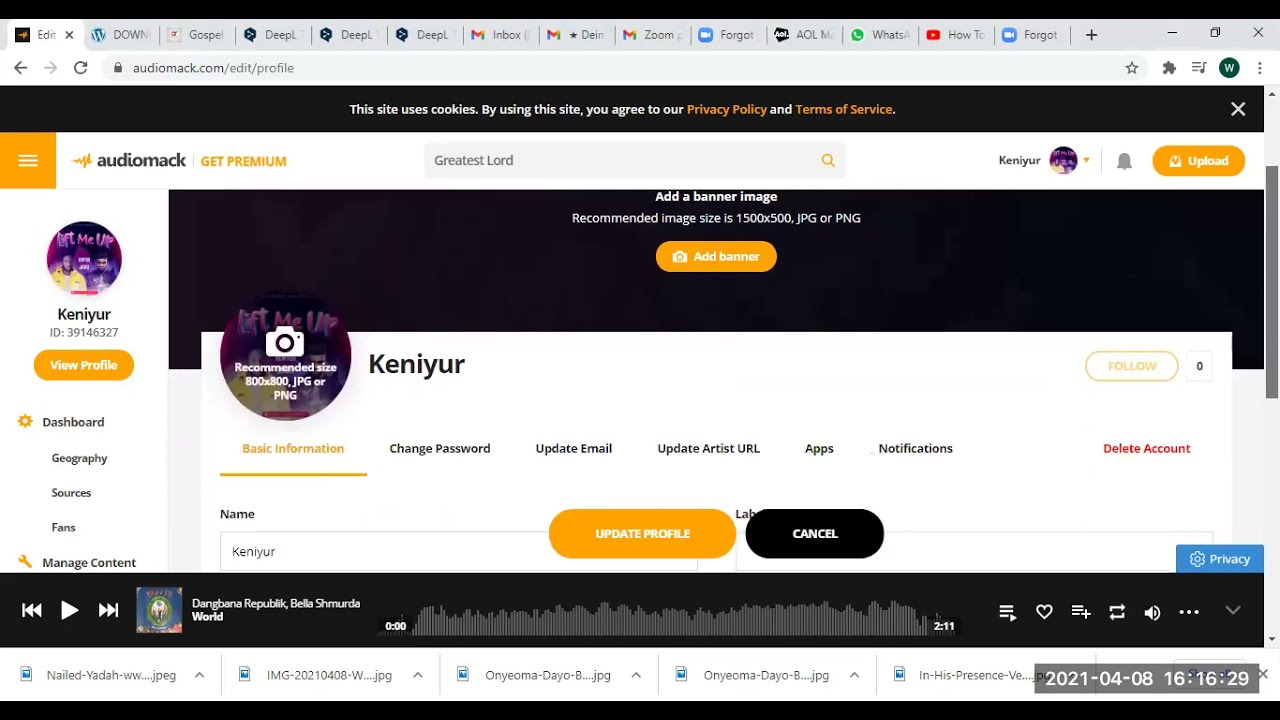The image captures a screenshot of the AudioMac website displayed on a computer screen, filled with various interactive elements and options. 

At the top of the browser, multiple tabs are visible, with the active tab showing "audiomac.com/edit/profile." The AudioMac logo is prominently located in the upper-left corner, accompanied by a yellow "Get Premium" button. In the center of the header, a search bar indicates a recent search for "Greatest Lord."

The user, identified as "Kenny Ur," is represented with a profile picture space. Adjacent to this, there is a gray notification bell icon and a yellow "Upload" button. On the left side of the screen, a sidebar displays "Kenny Ur, ID 39146327," along with several options: View Profile, Dashboard, Geography, Sources, Fans, and Manage Content.

Dominating the central part of the image is Kenny Ur's editable profile page, where the user can update their profile information and add a picture. Text fields are available to change the name, with options to "Update Profile" or "Cancel."

At the bottom of the screen, a black bar indicates a song currently playing: "World" by Deng Banna, Republic, and Bella Shmurda. Additionally, various media files, such as images or songs, are seemingly opened and displayed at the bottom of the browser.